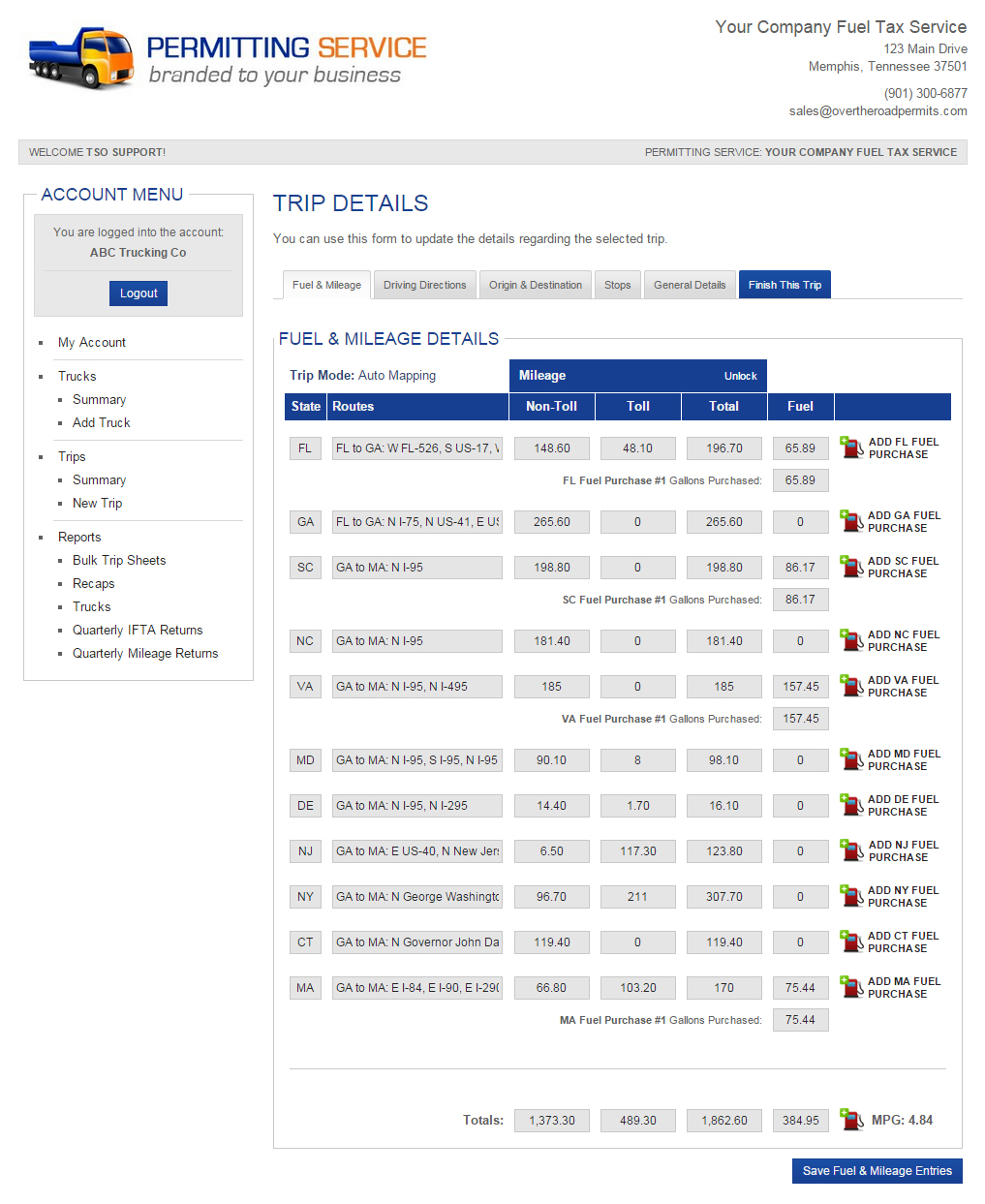**Descriptive Caption:**

This web page belongs to a permitting service branded to a business, recognizable by its distinctive dump truck logo. Positioned prominently at the top right, it displays the company name, "Your Company Fuel Tax Service," alongside the address: 123 Main Drive, Memphis, Tennessee, 37501. The contact details include a phone number, 901-300-6877, and an email address, sales@overtheroadpermits.com. 

Beneath this, a light gray box welcomes users to the support section, with the title "SO Support" and the subtitle "Permitting Service" prominently displayed. To the left of the page, the navigation menu shows that the user is currently logged in. The menu includes sections such as "Account," with options for "Trucks Summary" and "Add Truck," and a section for "Trips," featuring "Summary," "New Trip," "Reports," "Bulk Trip Sheets," "Recaps," "Quarterly IFTA Returns," and "Quarterly Mileage Returns."

The main content area features a detailed trip form, titled "Trip Details." Users can update details regarding their selected trip through various tabs, including "Fuel and Mileage," "Driving Directions," "Origin and Destination Stops," "General Details," and "Finish This Trip," the latter of which is the current focus. 

Under the "Fuel and Mileage Details" section, the page lists entries within a table bordered in dark blue. The entries are categorized by state, routes taken (both non-toll and toll), and fuel information. The totals for these entries are as follows: non-toll routes total 1,373.30 miles, toll routes total 488.90 miles, resulting in a combined total of 1,862.60 miles. The fuel consumption is recorded at 384.95 gallons.

This comprehensive layout ensures users can efficiently manage their permitting and fuel tax services, reinforcing the business’s commitment to streamlined, accurate service.